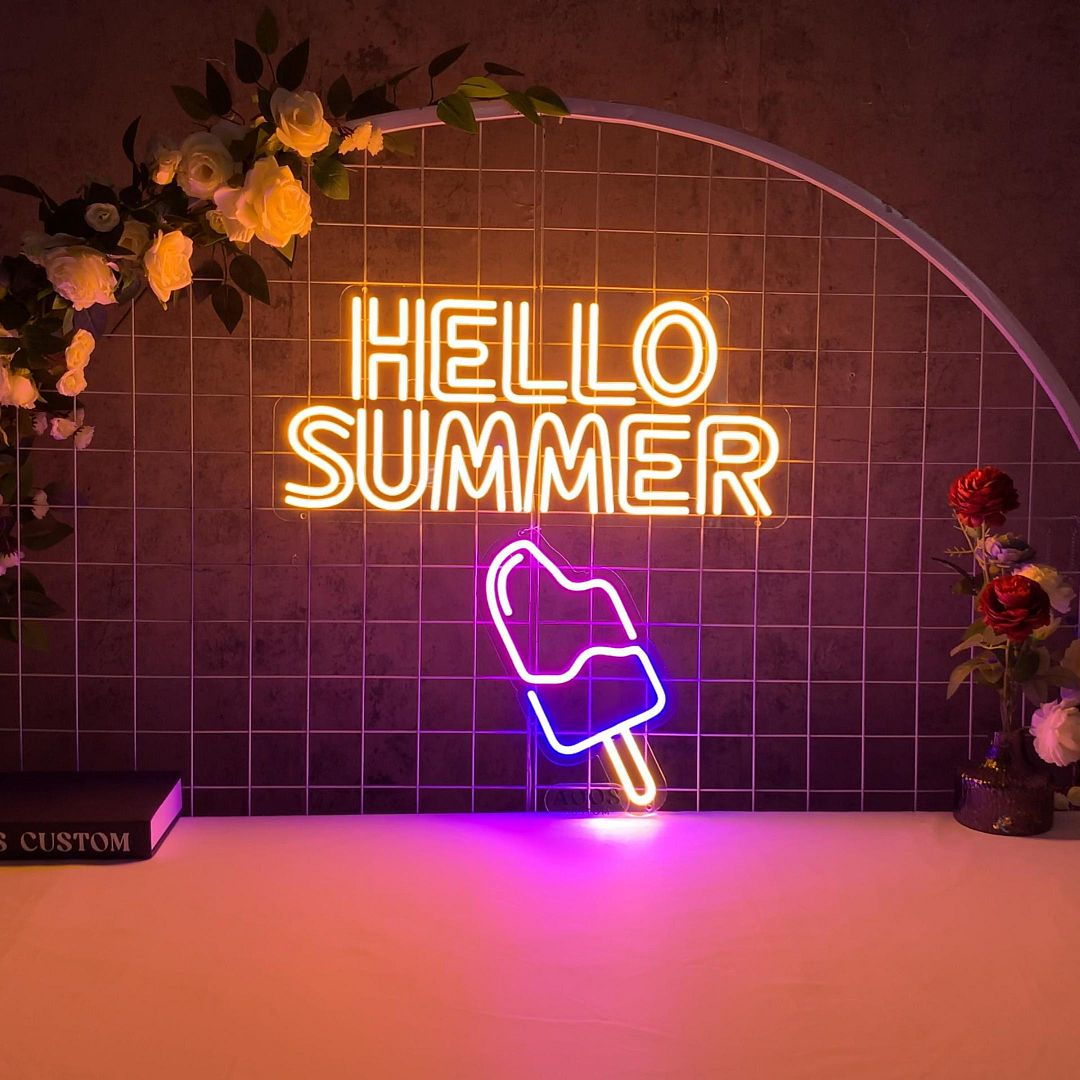This vertically rectangular, full-color photograph captures a vibrant, indoor scene under artificial light. The lower third of the image displays a white table or countertop with a partially visible hardcover book in the lower left corner, bearing the word "Custom." On the far right side, a bouquet of flowers with red, yellow, and white blooms adds a touch of nature.

Central to the photograph is a neon setup featuring an intricately detailed "Hello Summer" sign. This sign, highlighted in yellow light, is affixed to an arched, crisscross-patterned half-circle with a white border. Large, bright yellow flowers with green leaves adorn the upper left corner of the arch. Beneath the text, a neon popsicle, colored blue on the bottom and red with a bite taken out of the top, draws the eye with its vivid details. The background behind this neon display appears to be a textured or painted dark brown wall, enhancing the overall visual appeal of the scene.